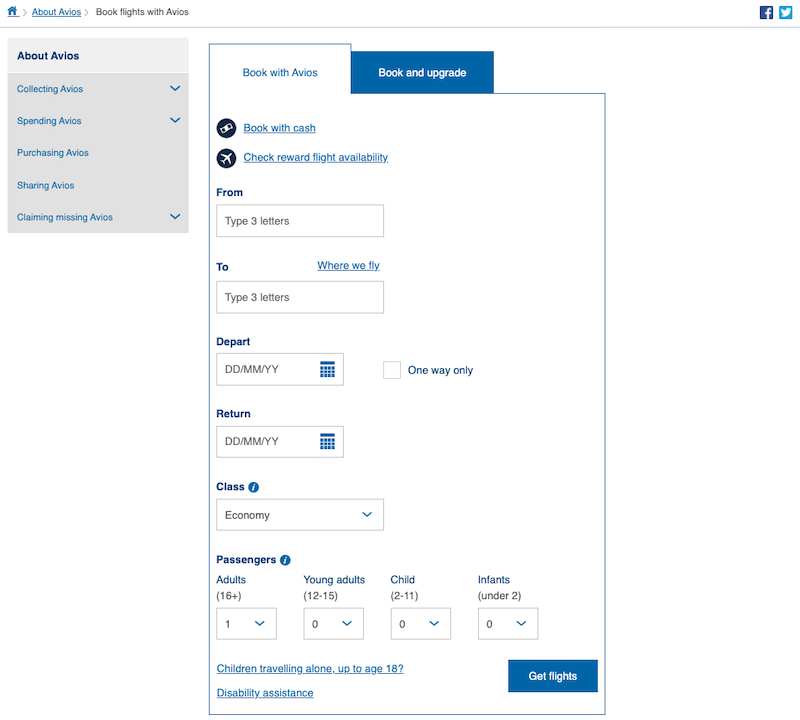The image depicts a section of a website or app designed for booking flights, with an emphasis on utilizing Avios points. 

In the upper left corner, there's a small blue home button, followed by text links for "About Avios" and "Book Flights with Avios." On the right side of the top header, social media icons for Facebook and Twitter are displayed.

Below the header, on the left side of the page, there is a gray square box titled "About Avios" with a set of options listed underneath: "Collecting Avios," "Spending Avios," "Purchasing Avios," "Sharing Avios," and "Claiming Missing Avios."

In the center of the page sits the main booking interface. Two tabs are visible at the top; the left tab, highlighted in white, reads "Book with Avios," while the right tab, in dark blue with white text, says "Book and Upgrade." 

The booking process directly below these tabs includes options such as "Book with Cash" and "Check Reward Flight Availability." Forms for entering flight details follow, labeled "From," "To," "Depart," "Return," and "Class of Flight." The "Economy" class is currently selected.